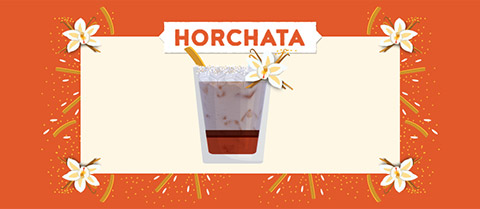The image depicts a vibrant poster or decorative piece centered around the popular Mexican drink, horchata. The main background is a warm orange color with speckled patterns resembling pollen. The focal point of the image is a centrally placed glass of horchata, featuring a yellow straw and adorned with a delicate white and yellow flower on the top right. The text "Horchata," prominently displayed at the top, is in an orange hue, reinforcing the theme. Surrounding the drink are four white flowers, positioned symmetrically in the upper left, upper right, bottom left, and bottom right corners, adding a harmonious floral touch. A subtle yellow box frames the drink, enhancing its visual appeal. The border of the image is thick and red, with floral accents in the corners and white and gold leaves extending toward the center, likely intended to create a decorative and inviting kitchen artwork feel. The design intricacies suggest careful attention to detail in the flowers and overall presentation, making it both attractive and culturally resonant.